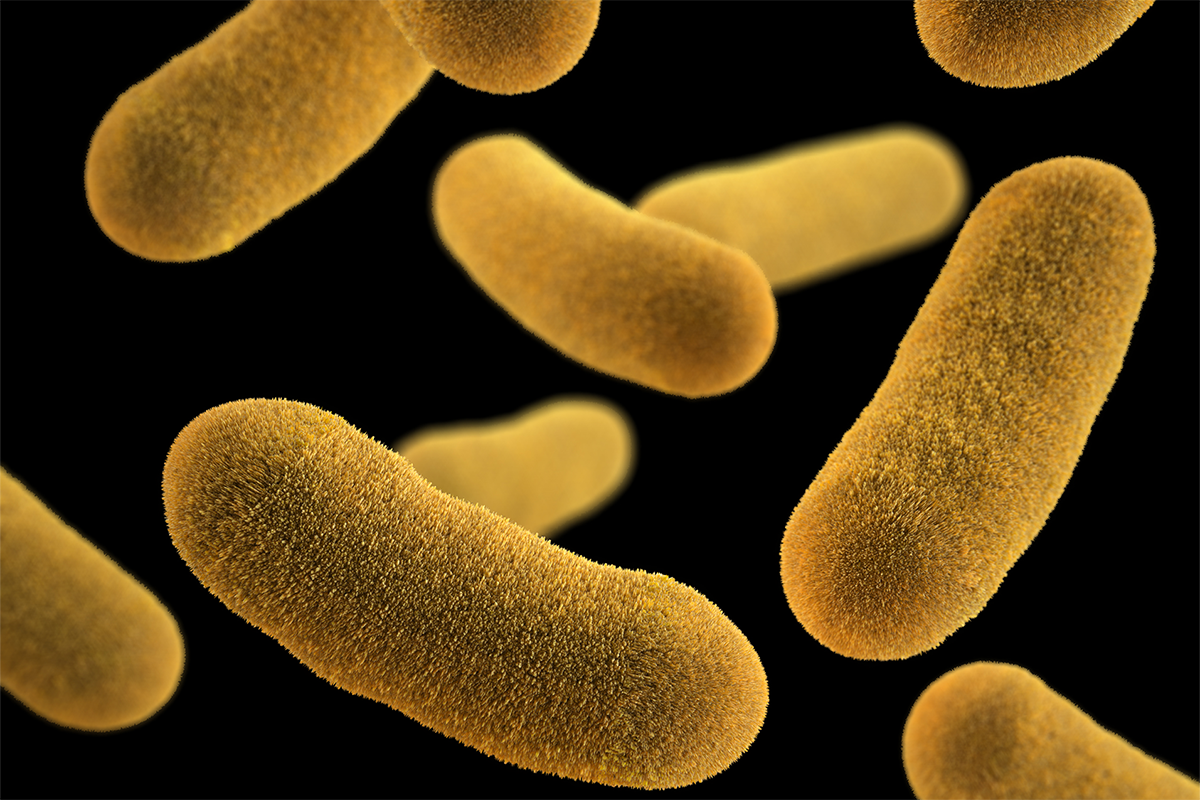The image depicts a highly detailed photograph, possibly taken through a microscope, showcasing around nine or ten floating, unicellular organisms against a completely black background. These organisms bear a striking resemblance to Cheetos, with a cylindrical, round shape and a grainy, powdered texture reminiscent of a short, hairy surface. The objects are vividly orange and seem to be suspended in mid-air, with no discernible pattern in their arrangement; they're randomly oriented in various directions, with some appearing more blurred than others. The overall scene creates an intricate and visually striking representation, alternately interpreted as magnified food items like Cheetos, corn on the cob, or potatoes, or as microscopic bacteria or molecules.